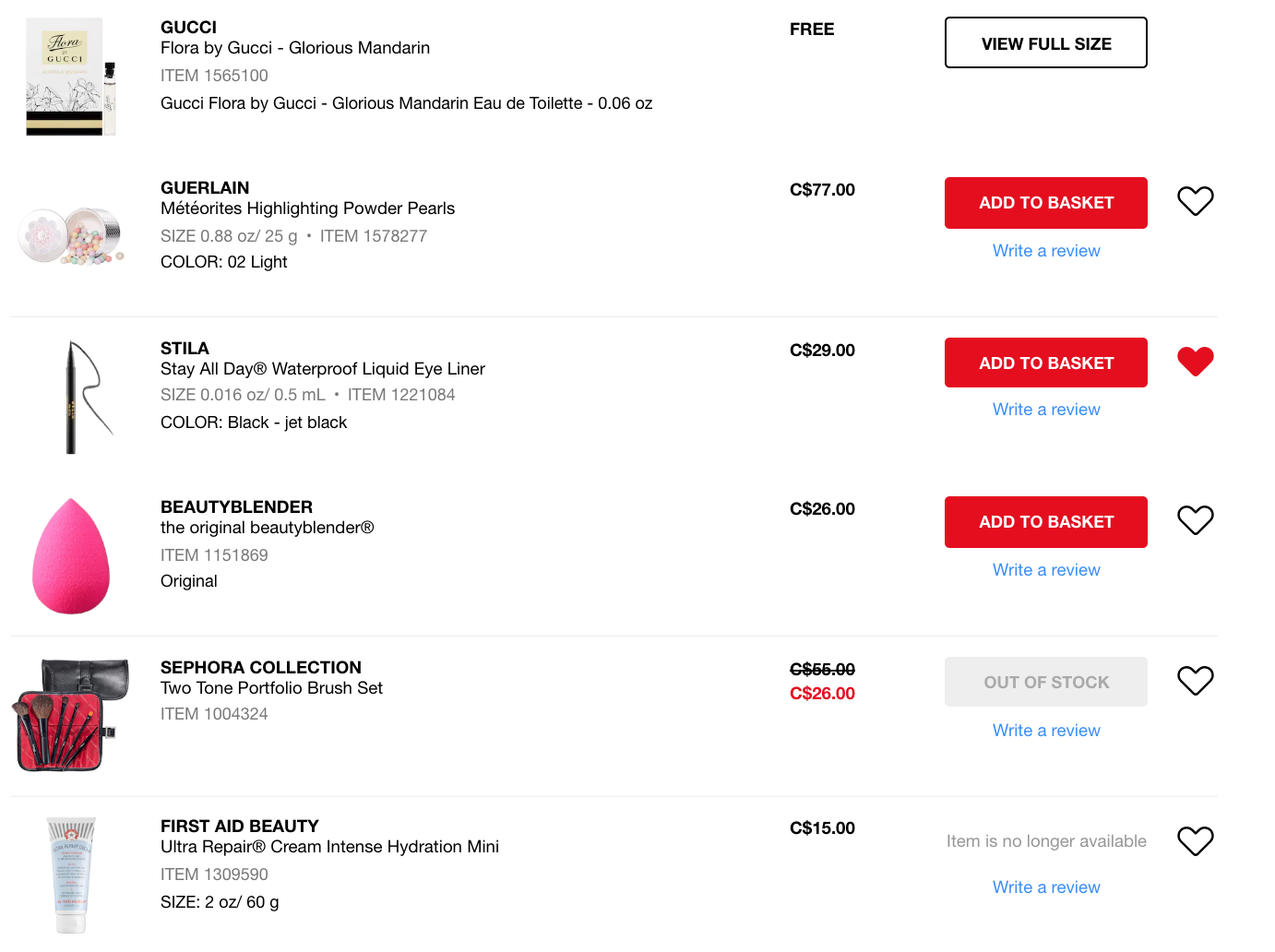This image is a screenshot from an e-commerce website, likely Sephora, based on the content displayed. The background is white, and neither the header nor the footer is visible, obscuring the exact identity of the website.

On the left side of the image, there is a detailed list of cosmetic products, each accompanied by an image:

1. **Gucci Flora by Gucci**
   - Image: An elegant bottle of perfume.
   
2. **Guerlain Meteorites Highlighting Powder Pearls**
   - Image: A luxurious container housing multicolored powder pearls.
   
3. **Stila Stay All Day Waterproof Liquid Eyeliner**
   - Image: A sleek, dark pencil-like eyeliner.
   
4. **Beauty Blender**
   - Image: A large, pink teardrop-shaped sponge.
   
5. **Sephora Collection Two-Tone Portfolio Brush Set**
   - Image: A black cosmetic bag with a red lining, containing a series of makeup brushes.
   
6. **First Aid Beauty Ultra Repair Cream Intense Hydration Mini**
   - Image: A white tube with small, unreadable fonts.

On the right side, aligned with each product, there is pricing information and availability:
- **Gucci Flora by Gucci**: Price available, with an "Add to Basket" button in a red rectangle with white font.
- **Guerlain Meteorites Highlighting Powder Pearls**: Price available, with "Add to Basket" button.
- **Stila Stay All Day Waterproof Liquid Eyeliner**: Price available, with "Add to Basket" button.
- **Beauty Blender**: Price available, with "Add to Basket" button.
- **Sephora Collection Two-Tone Portfolio Brush Set**: Marked as "Out of Stock."
- **First Aid Beauty Ultra Repair Cream Intense Hydration Mini**: Labelled as "Item is no longer available."

This detailed layout provides a clear snapshot of the available, out-of-stock, and no longer available cosmetic products on the website.